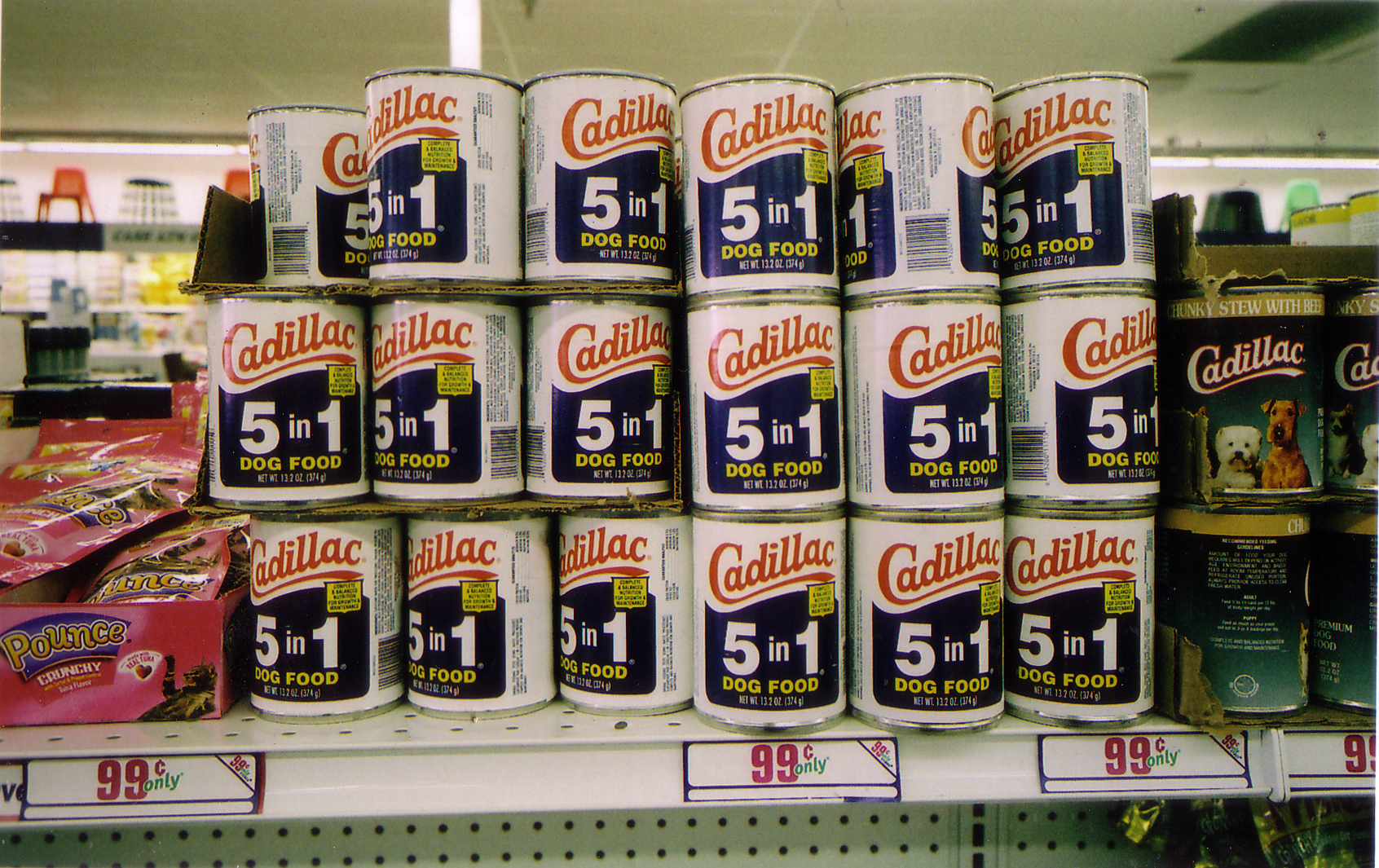The image depicts a display shelf in a grocery store, specifically a $0.99 store, with an assortment of pet products. The focal point is on various cans of Cadillac dog food. The shelf itself is white and features peg holes for hanging items. Prominent on the shelf are four white price labels each displaying "$0.99 only" in red, with the word "only" in green, and a small triangle in the corner repeating the price.

In the center, there is a can of Cadillac dog food with a simple white and silver design. The top of the can has 'Cadillac' written in cursive red, followed by a blue section with "5 in 1" in white letters, and below that, "dog food" in yellow. The exact net weight is unclear, but it's either 133 ounces or 13.3 ounces. 

To the right of this can is another variety of Cadillac dog food in a bluish-green labeled can marked "Chunky Stew with Beef." This can features an image of two dogs, an Airedale and possibly a Bichon Frise, with "Cadillac" written in white cursive.

Also on the right side of the display is a product labeled "Pounce Crunchy," which appears to be a cat treat. The packaging is pink, featuring an image of a playful cat on its back near the treats.

In the background, above the shelf, the white ceiling panels and additional store items are visible, contributing to the setting of an organized store environment.